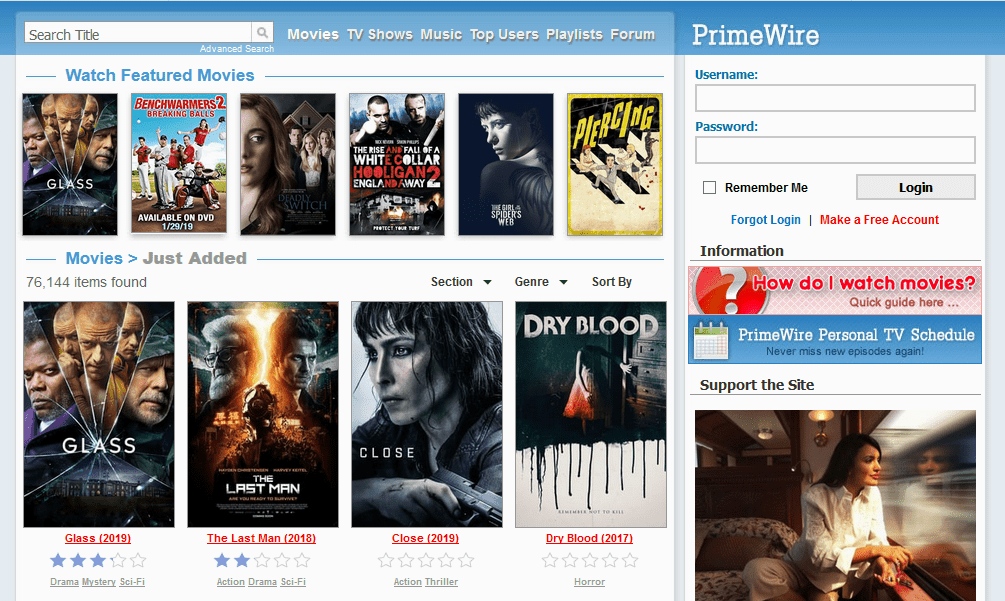The image depicts the homepage of the Prime Wire website. On the right side, you'll see the Prime Wire logo alongside input fields for the username and password, both of which are highlighted in blue. These long rectangular boxes are where users enter their login details. Below this, there is an option to check a "Remember Me" box for saving login information, along with a "Login" button. There is also a "Forgot Login" link and an option to create a free account.

At the top of the page, a search bar allows users to look up titles, movies, TV shows, music, top users, and playlists, with all these categories displayed in blue. Below the search bar, there is a section featuring movies such as "Glass," "Benchwarmers," "White Collar," "Pure Clean," "Dry Blood," "Close," and "The Last Man." The website boasts a collection of 76,144 items.

Users can sort content by genre and rating. The movies "Glass," "The Last Man," "Close," and "Dry Blood" have their star ratings displayed, with "Glass" receiving three stars, and "The Last Man" receiving two stars. "Close" and "Dry Blood" currently have no ratings. The genres listed include Drama, Mystery, Action, Thriller, and Horror. 

The background of the website is predominantly white, with blue highlights throughout. A feature called "Prime Wire Personal TV Schedules" allows users to create their own schedule guides. Additionally, there is a support section depicted by an image of a Caucasian woman with long hair, wearing a white shirt and khaki pants, sitting on a bed and looking out of a window.